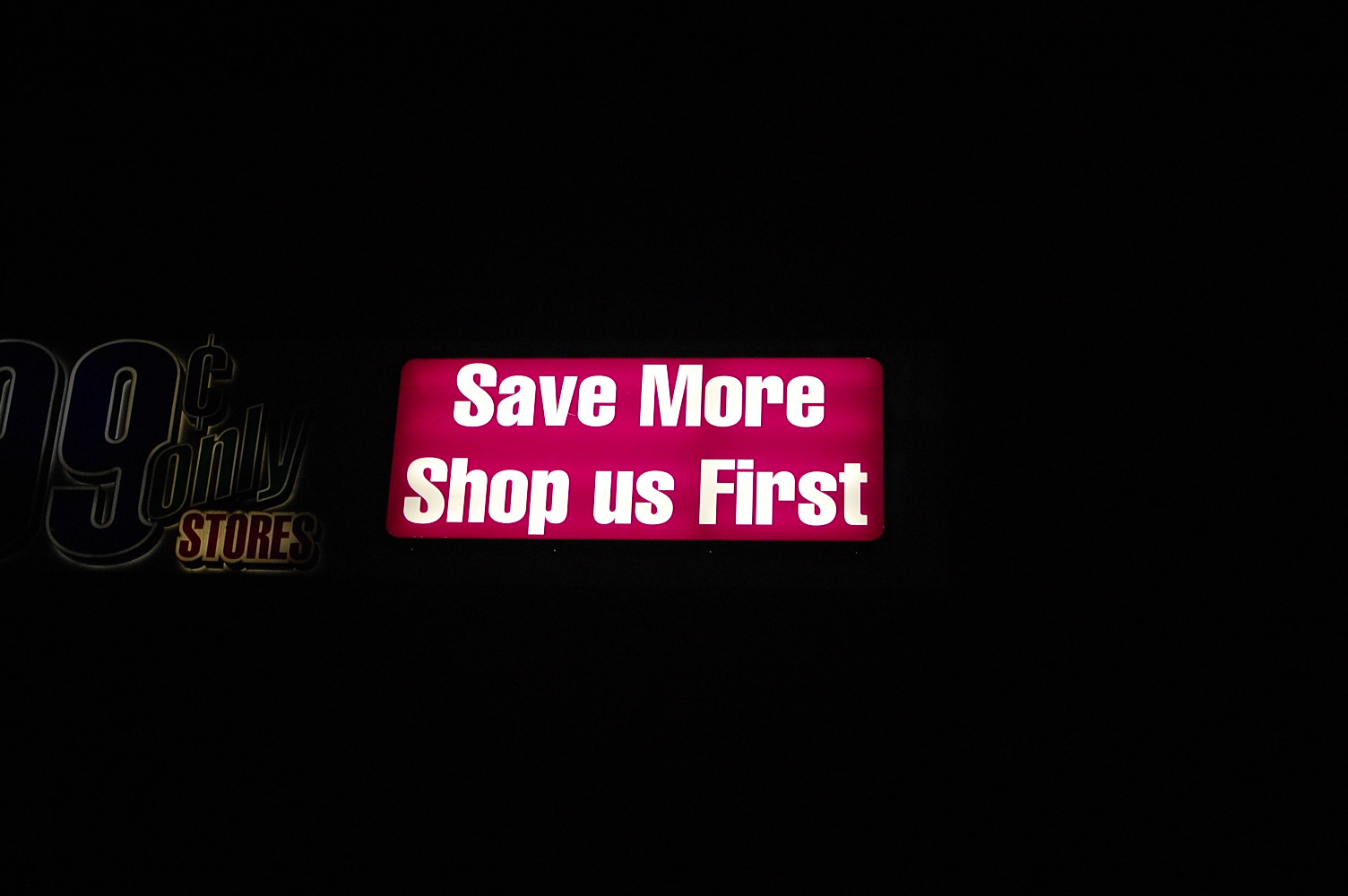This photograph, taken at night, features a store's exterior with a predominantly black background, making the signs stand out distinctly. On the left-hand side, there is a dimly lit sign that shows the words "99 Cent Only Stores." The text "Stores" is written in red letters on a yellow background section, though overall, the sign is faint and not well illuminated, making it harder to notice. Dominating the center of the image is a brightly lit rectangular red sign adorned with light bulbs, drawing significant attention. This sign reads "Save More" at the top in white text, with each word capitalized. Below, also in white text and capitalized, are the words "Shop." Underneath that is "us" in lowercase letters followed by a capital "F" leading into the word "First," completing the phrase "Shop us First." This vibrant central sign contrasts sharply against the dark background, making it the focal point of the image.